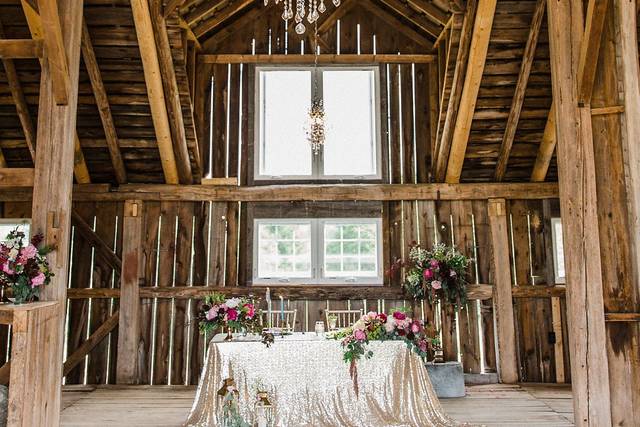The image depicts a beautifully decorated wedding setup inside a pristine, wood-stained farmhouse or barn. The venue is strikingly clean and boasts a rustic yet elegant ambiance. Prominently featured is a table for two, intended for the bride and groom, draped in a long, white lacy tablecloth that cascades to the floor. Behind the table are two white high-back chairs, adding to the sophisticated setting. The table is adorned with a blue candle, contrasting gracefully with various vibrant floral arrangements in shades of dark purple, maroon, white, and carnation pink, both on the table and flanking it on either side.

In the background, a white-framed window is featured prominently, flanked by two smaller side-by-side windows below it. Above, a chandelier adds an elegant touch, casting soft light across the room. A hanging bouquet or plant dangles subtly from the ceiling, adding depth to the decor. To the left side of the table, a small wooden ledge hosts more floral arrangements, completing the picturesque setup. The overall scene is a harmonious blend of rustic charm and elegant details, perfectly suited for a wedding celebration.